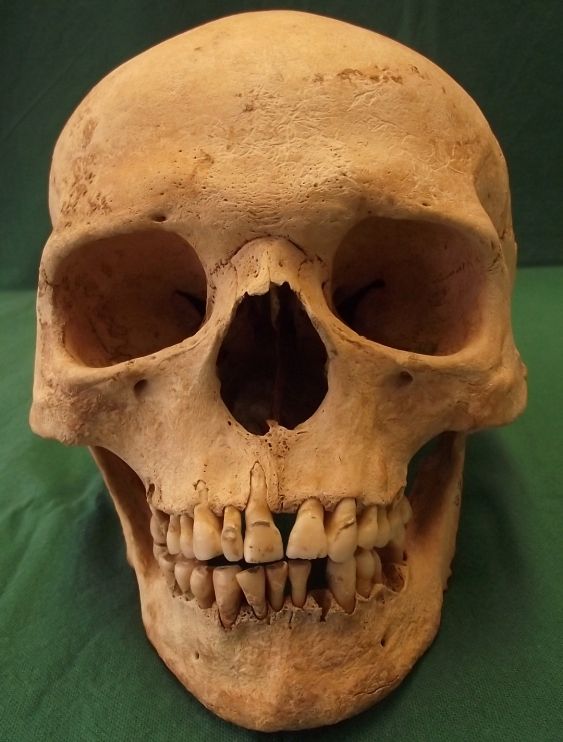The image depicts an excavated skull, likely unearthed after being buried for an extended period. The skull, devoid of any skin or flesh, reveals intricate anatomical details. Its color is a brownish beige rather than a typical white. The eye sockets and nasal cavity appear hollow, as do the cheek areas, showing just the cheekbones. The dental structure is visible, showcasing where the roots of the teeth once were. Despite some minor markings, the top of the skull remains intact, with no visible cracks. Notably, there are two small indentations on either side of the chin, possibly indicating the presence of dimples, along with two larger holes beneath the eye sockets. The background consists of a green fabric with a darker green backdrop, upon which the skull is positioned.